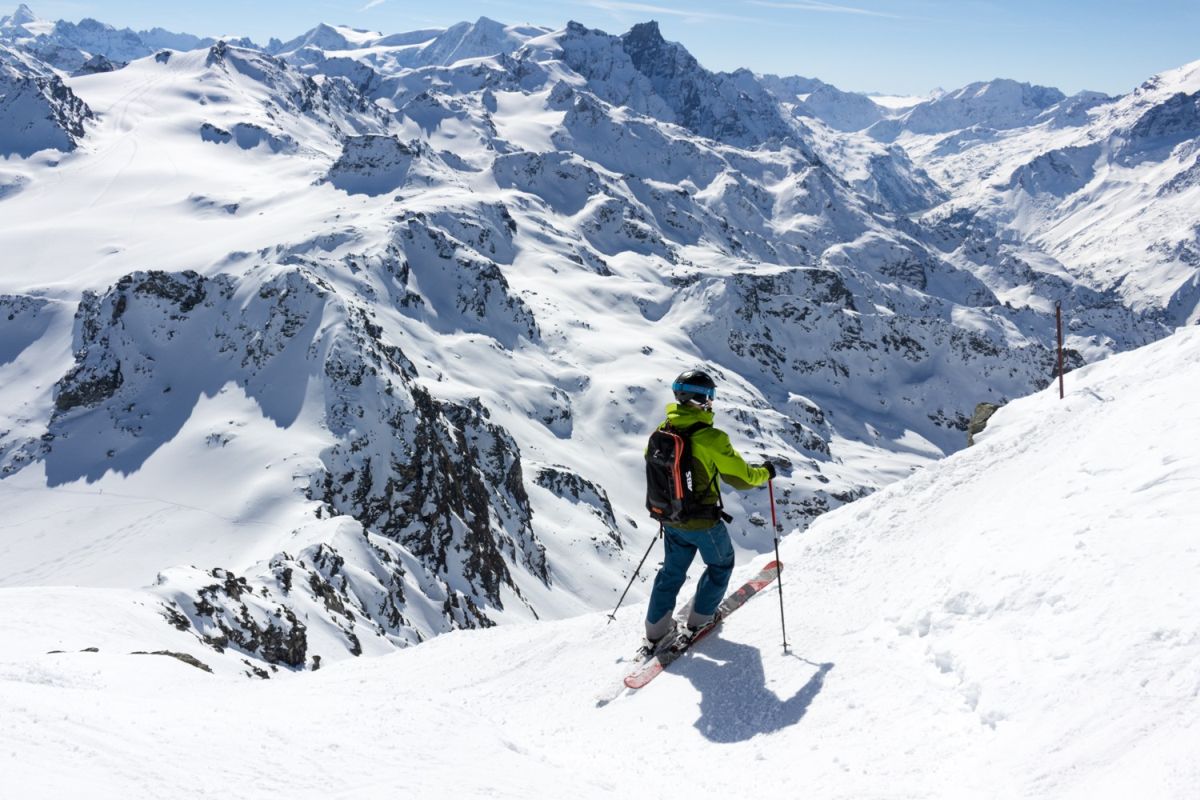In this stunning photograph, a solitary skier is captured mid-mountain, facing the upper right corner of the frame. He stands on a snowy slope adorned in a distinctive lime green jacket and blue ski pants, complemented by a black helmet. A knapsack rests on his back, and he grips red ski poles, matching his red skis. The scene is bathed in brilliant natural light, reflecting off the pristine white snow, with a clear blue sky dotted with white clouds overhead. The vast, majestic mountain range stretches out before him, covered in snow and untouched by any other presence, emphasizing the serene solitude and breathtaking beauty of this high-altitude adventure.